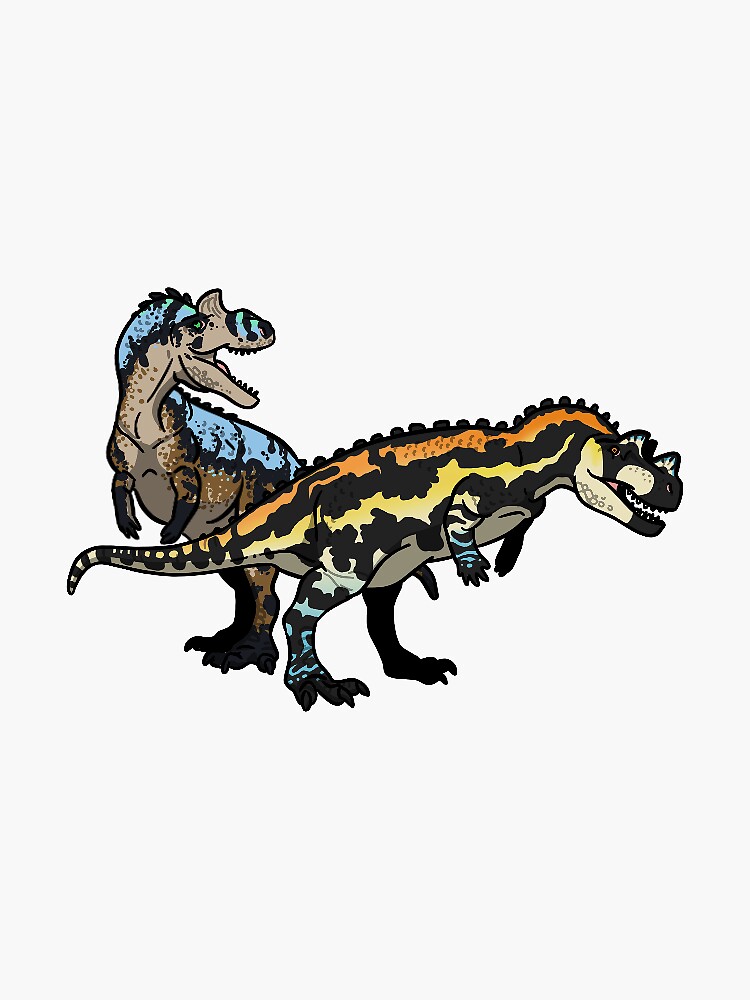The image is a colored drawing, likely intended for a children's book, featuring two cartoonish Tyrannosaurus rex-like dinosaurs on a clear white background. Both dinosaurs have small, stubby arms and horn-like humps on their heads, resembling a T-Rex but with unique features. The dinosaur in the background has a predominantly sky blue coloration along its nose, neck ridge, and back, with dark brown hands and feet, and a gray underbelly. The dinosaur in the foreground showcases a vibrant orange and yellow gradient along its back and nose, with blue accents on its legs and dark brown skin. The two dinosaurs are positioned one behind the other, adding depth to the simple yet colorful illustration.